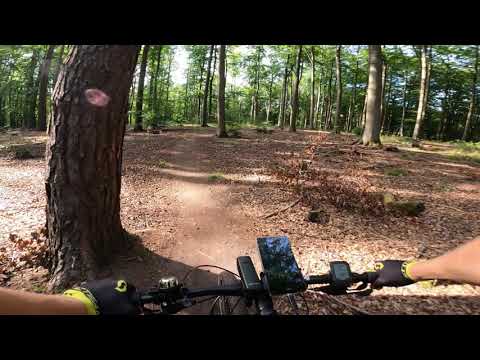In this high-definition, horizontally rectangular image framed by dark borders on the top and bottom, we find ourselves in a forest clearing, not densely packed with trees but rather a wide-open area with sparse tree cover. Dominating the left foreground is the trunk of a very large tree, notable for its oval spot devoid of bark, possibly used for sap extraction.

Lying at the foot of this tree is a bicycle on its side, clearly visible. On the right side of the image, there's a hand—belonging to a white male wearing yellow and black gloves—either setting the bicycle down or preparing to pick it up. This person is also seen gripping the handlebars of the bike, which is equipped with a smartphone holder in the center, the phone illuminated, with a speedometer to its right and some controls to the left.

The middle of the image features a muddy, brown, flowing river with debris floating on its surface, which serves as the natural boundary to more forested land in the background. The riverbanks are muddy, giving way to patches of green grass or weeds and numerous trees with lush green leaves. The overall color palette of the photo includes earthy browns, vibrant greens, touches of yellow from the gloves, and patches of blue sky peeking through the partly cloudy sky, highlighting the sunlight filtering through the trees.